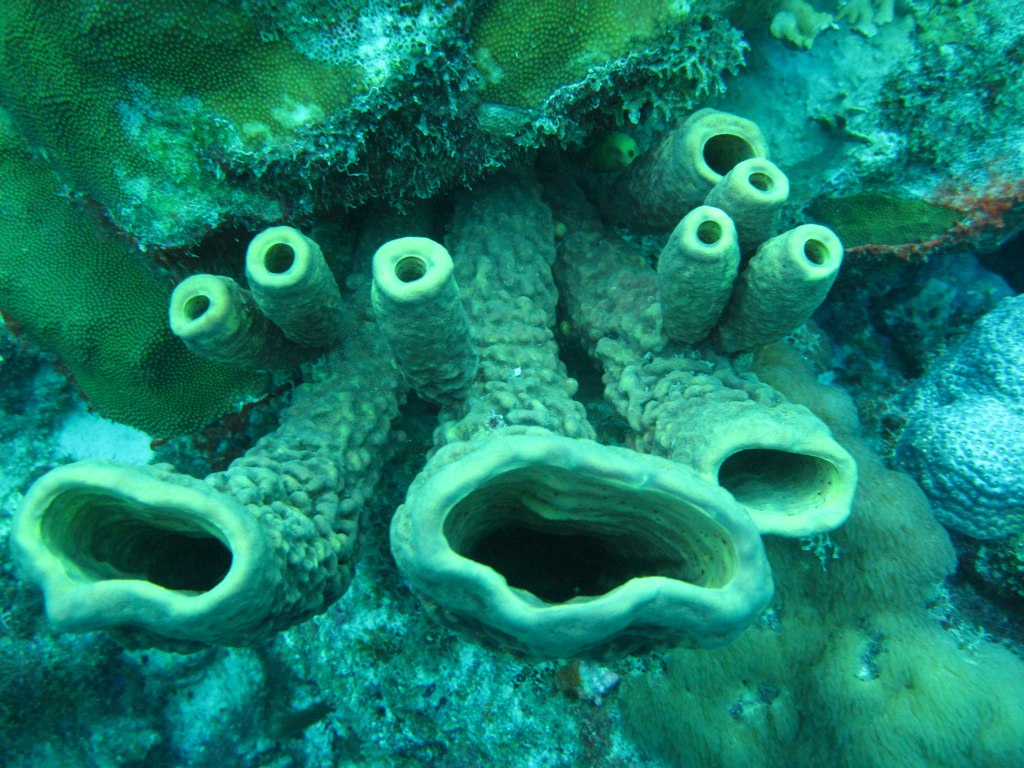This underwater photograph captures a vibrant piece of the seabed, approximately 20 feet below the surface, where sunlight still penetrates, casting a turquoise green-blue hue over the scene. Dominating the image are intriguing coral formations resembling tubes with a snout-like appearance; notably, there are six smaller tubes, with three each on the left and right, and three larger, elongated ones extending across the middle to the left. The coral exhibits a greenish hue, likely an effect of the lighting and the water. Additionally, there is a large, jagged sponge characterized by small dots visible in the background, along with an array of green algae that varies in texture and height throughout the scene. This lush bed of marine life includes patches of flat, mold-like algae and taller varieties on the right, interspersed with slight touches of red, adding to the intricate tapestry of colors.